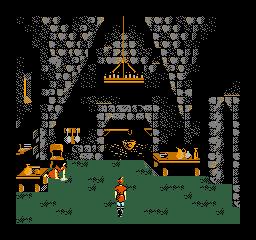This image, a screen capture from a retro 90s-style video game, depicts a scene set inside a castle room with simpler, cartoon-like graphics. In the center of the room, a character with their back to the viewer is clad in an orange tunic or one-piece outfit, complemented by a brown hat, black boots, white arms, and blue legs. The character stands on a green carpet that covers about a third of the floor area. The room's walls are composed of stone textures with a mixture of black and gray highlights.

The room features wooden tables on each side, adorned with various items including dishes and pictures. A wooden chair is positioned to the left, while the back wall is dominated by a large fireplace, complete with a cooking pot suspended from a stick. A chandelier, hanging from the ceiling, is an eye-catching feature, boasting multiple candles along its length.

The atmosphere is accentuated by the intricate details: a big, square table to the right with additional items, and a peculiar black spot on the right wall, possibly indicating another entrance. The overall scene is framed by a black border, enhancing the nostalgic aesthetic of the game.